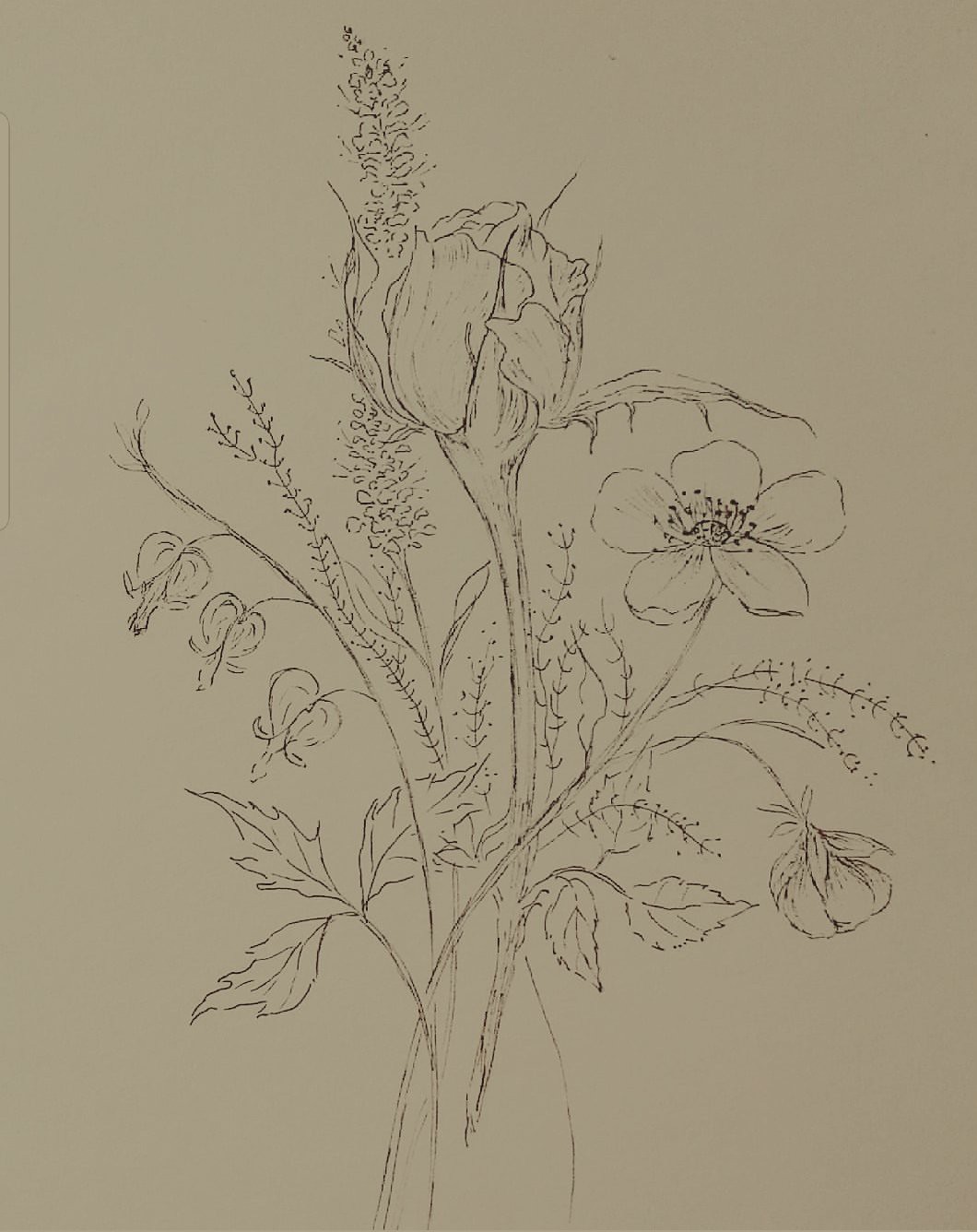This detailed pencil sketch on a white piece of paper showcases a diverse collection of floral elements arranged in a vertical composition. At the left of the sketch, we see flowers growing on a gracefully arched stem, coupled with a small leafy design near the bottom left. In the center, a prominent rose takes the spotlight with its detailed petals, flanked by smaller wildflowers, one of which resembles a blue bonnet or bluebell. Ascending upwards from the middle are several twigs adorned with tiny, intricate leaves. To the right, a charming daisy with five rounded petals and a distinct dark center, rich with filaments, contrasts against a background element that looks like a cat's tail or foxtail, characteristic of wild country flora. The entire image is rendered in black and white, enhancing the detailed pen or pencil work and making it challenging to precisely identify all flower species, but suggesting a collection of at least five different types. The absence of an artist’s signature hints at the humble yet skilled hand that created this intricate piece.